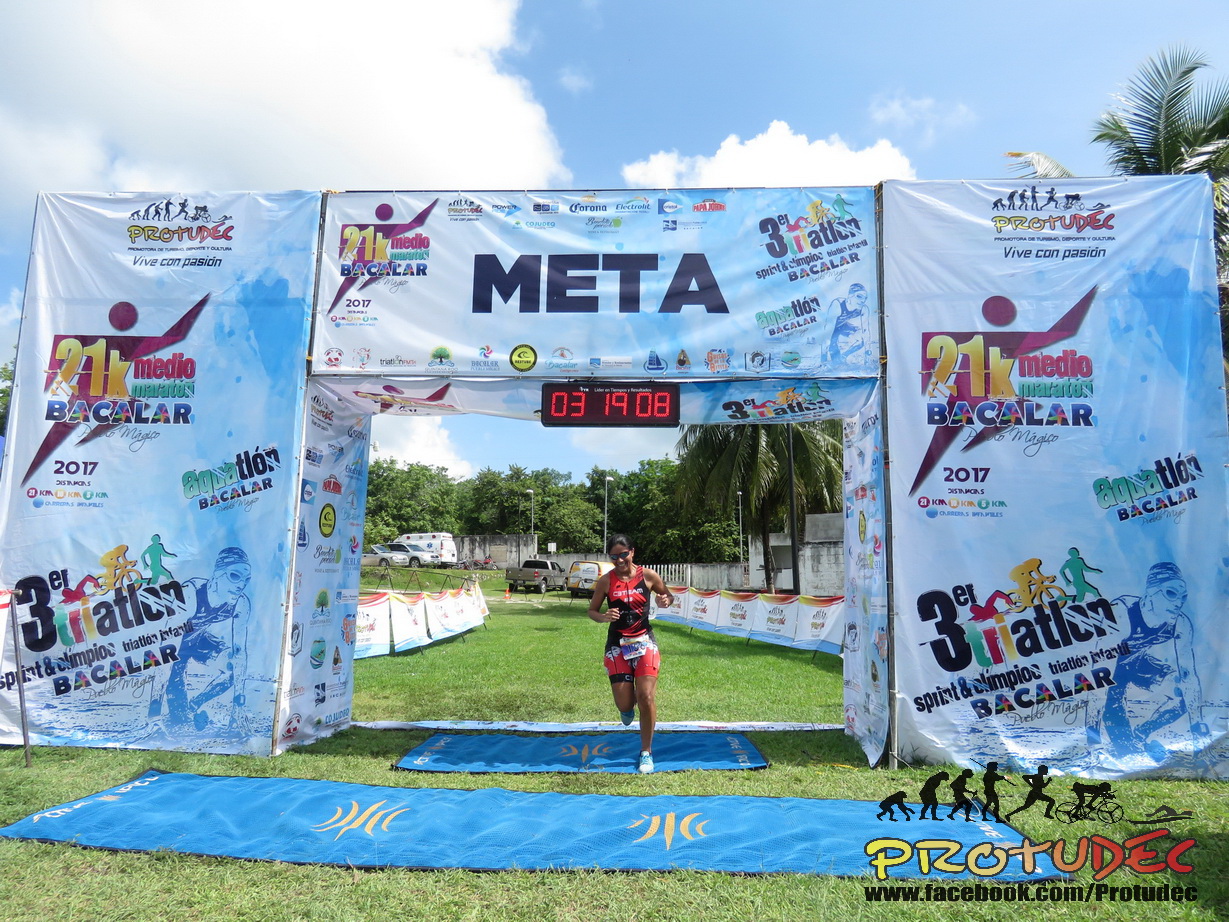This detailed photograph captures a young, possibly Asian, Indian, or Latino woman, crossing the finish line of a triathlon. She has long dark hair pulled back into a ponytail and wears dark black sunglasses. Dressed in a red, black, and white tank top that seamlessly blends with her matching spandex shorts—possibly a one-piece outfit—she has her runner's number displayed around her waist. Behind her, a large patch of green grass is visible, populated by parked cars, trucks, and an ambulance, signify the event's broad support and logistics.

The finish line is an impressive setup consisting of two tall pillars adorned with various signs and logos related to the triathlon. Suspended between these pillars is a banner prominently displaying the word "META" in black letters, alongside numerous other texts and images. Notable mentions include "21K Media Marathon Baccalaureate 2017" and "3er Triathlon Spirit and Olympio Olympic Triathlon Baccalaureate." Above her head, a ticker clock on the banner displays her finish time, emphasizing the culmination of her endurance effort. The ground she runs on is blue carpet laid over the grass, further dignifying the race’s conclusion. The sky overhead is blue with scattered clouds, framing a clear day for the event.